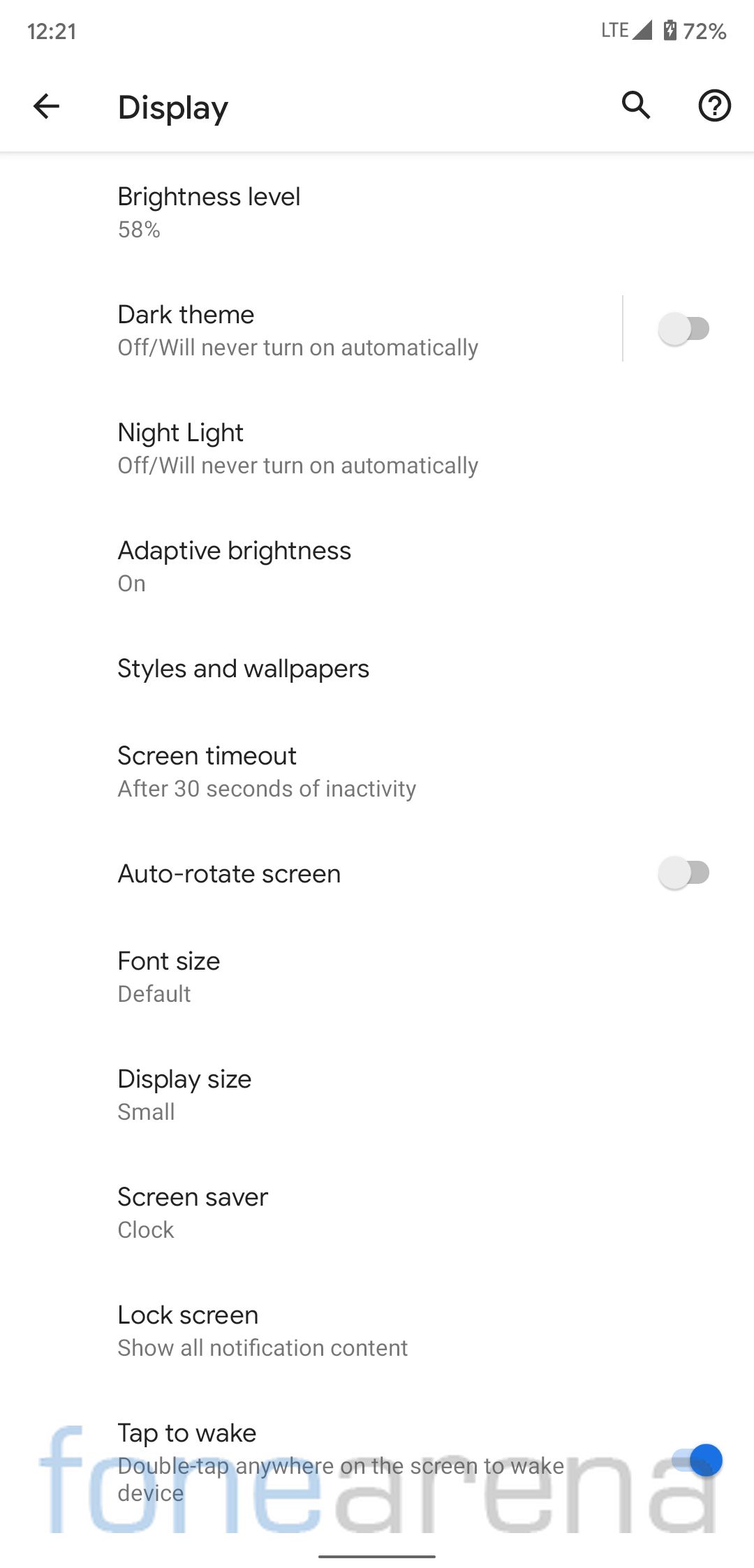Screenshot of a cell phone settings screen at 12:21 (AM/PM not specified). The phone is connected to an LTE network with full signal strength and has a 72% battery charge. At the top, the navigation bar features a back arrow, the word "Display," a magnifying glass icon, and a circle with a question mark.

The details of the "Display" settings are as follows:
- Brightness level is set at 58%.
- Dark theme is off and will never turn on automatically (toggle switch is off).
- Night Light is off and will never turn on automatically.
- Adaptive brightness is enabled.
- Styles and wallpapers section is present but currently empty.
- Screen timeout is set to activate after 30 seconds of inactivity.
- Auto-rotate screen feature is turned off.
- Font size is set to default.
- Display size is set to small.
- Screensaver is set to display the clock.
- Lock screen will show all notification content.
- "Tap to wake" feature is enabled, allowing the device to wake up with a double-tap anywhere on the screen.